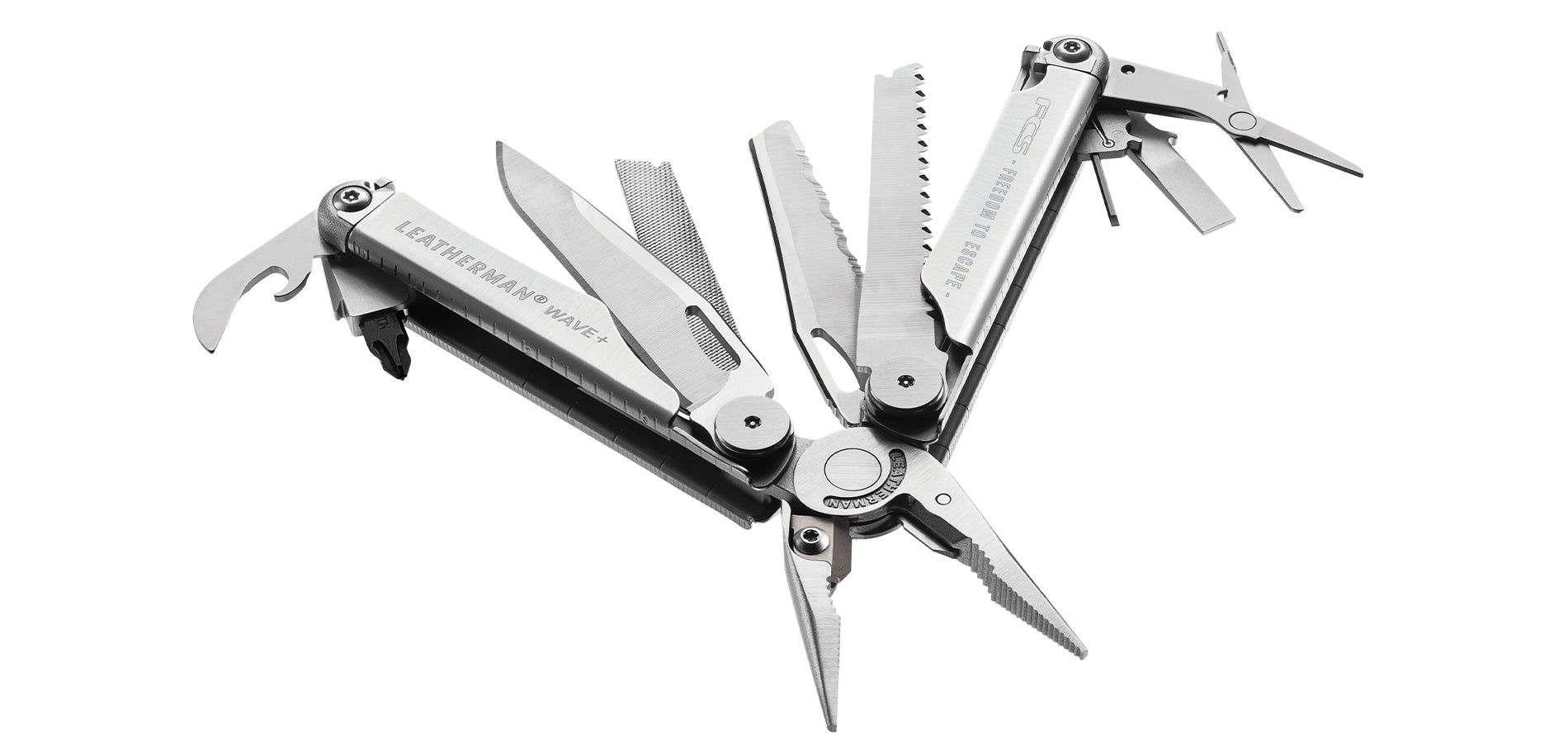This image prominently features a Leatherman Wave Plus multi-use tool, showcasing its versatility and utility. The device, made entirely of silver metal except for the star-shaped screwdriver bit, displays an array of functionalities typical of a high-quality multi-tool. Open to reveal its components, it includes pliers at the center, surrounded by various tools such as a flathead screwdriver, a star screwdriver, a knife, a file, a bottle opener, scissors, and two saws—one serrated and one non-serrated. Additionally, there is a small lock pick and a pair of mini clippers embedded in its design. On one side of the tool, the brand name "Leatherman Wave Plus" is precisely etched, while the other handle bears the phrase "Freedom to Escape FCS," enhancing its appeal as a reliable tool for a wide range of tasks.